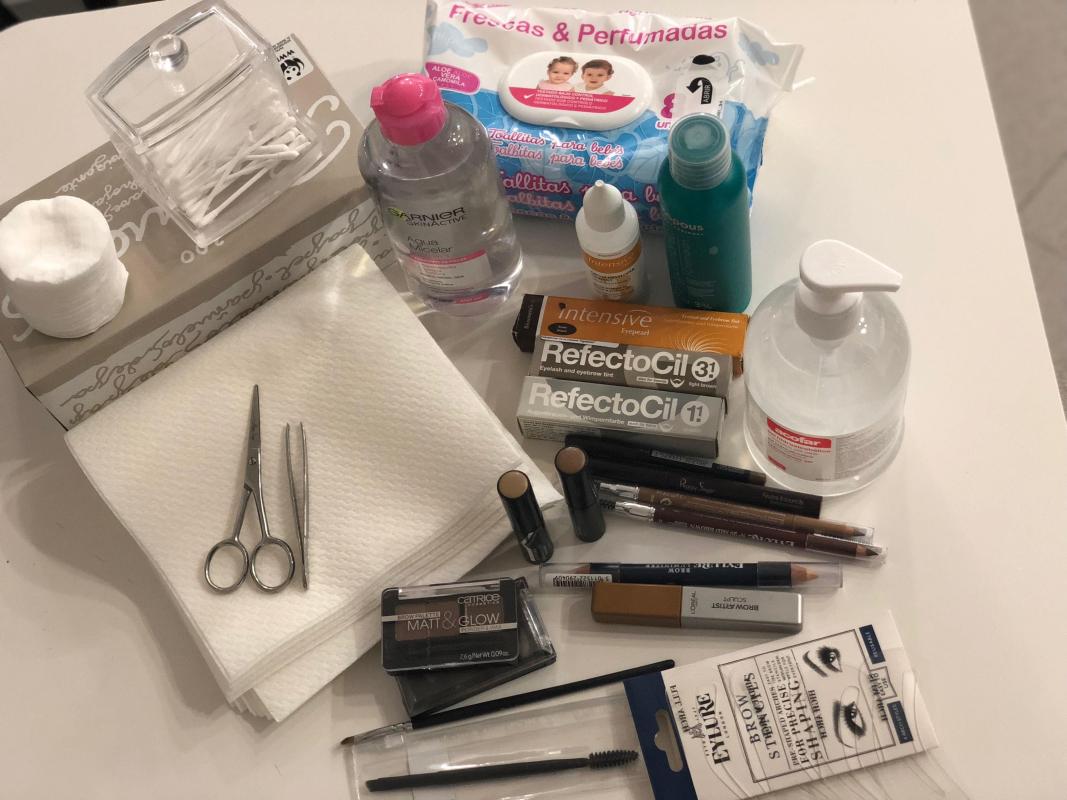An overview shot of a meticulously arranged bathroom countertop laden with an array of health and beauty products. On the left side, a neatly stacked pile of white napkins is topped with a pair of tweezers and a small pair of handled scissors, indicating a focus on grooming tools. Adjacent to this, a stack of flat cotton pads is perfectly aligned, while a clear plastic square container brimming with Q-tips stands nearby. Below these items, a large bottle of Garnier eye makeup remover dominates the scene, flanked by a plastic package of baby wipes adorned in pink and blue hues. The rest of the countertop features a diverse collection of lotions, medicinal products, and makeup essentials. Eyeliners and eyebrow pencils mingle with various soaps, while a pristine mascara wand adds a finishing touch to the display. The organized chaos suggests a deliberate attempt to showcase a well-rounded selection of beauty aids.